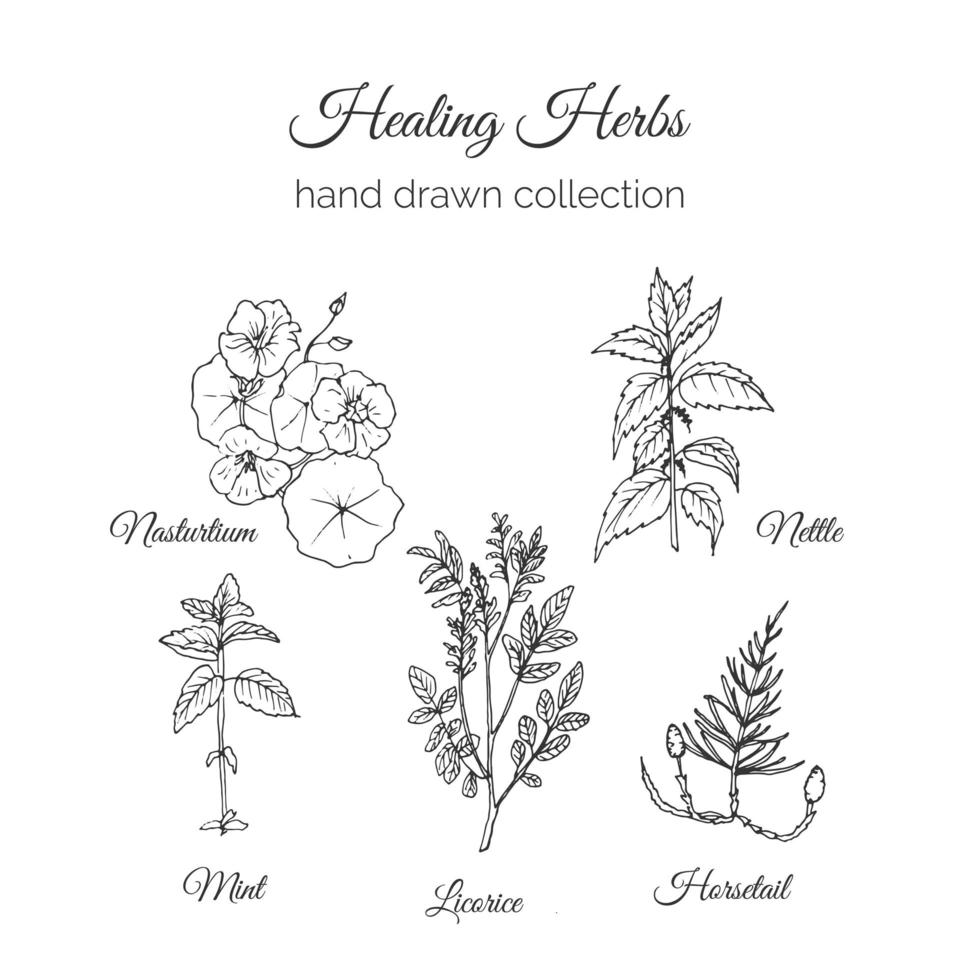The image features a collection of five meticulously hand-drawn herb illustrations, rendered entirely in black and white, without shading or intricate detail. At the top of the image, the words "Healing Herbs" are elegantly scripted, while beneath this, "Hand-Drawn Collection" is written in plain block text. Each herb’s name is labeled in cursive script. 

On the top row, the leftmost image showcases a nasturtium with its characteristic round, circular flowers. Beside it is an illustration of nettle, identifiable by its stalk and teardrop-shaped leaves with serrated edges. 

On the bottom row, starting from the left, there is a depiction of mint, distinguished by its smooth-edged leaves and thinner stalk. The middle illustration features the licorice plant, which has a central stalk branching into smaller leaves. The final image on the right is of the horsetail plant, characterized by multiple buds and conical, almost flowering blooms resembling a pine tree structure.

The overall scene, set against a clean white background, looks as though it might be a page from a vintage botanical book.